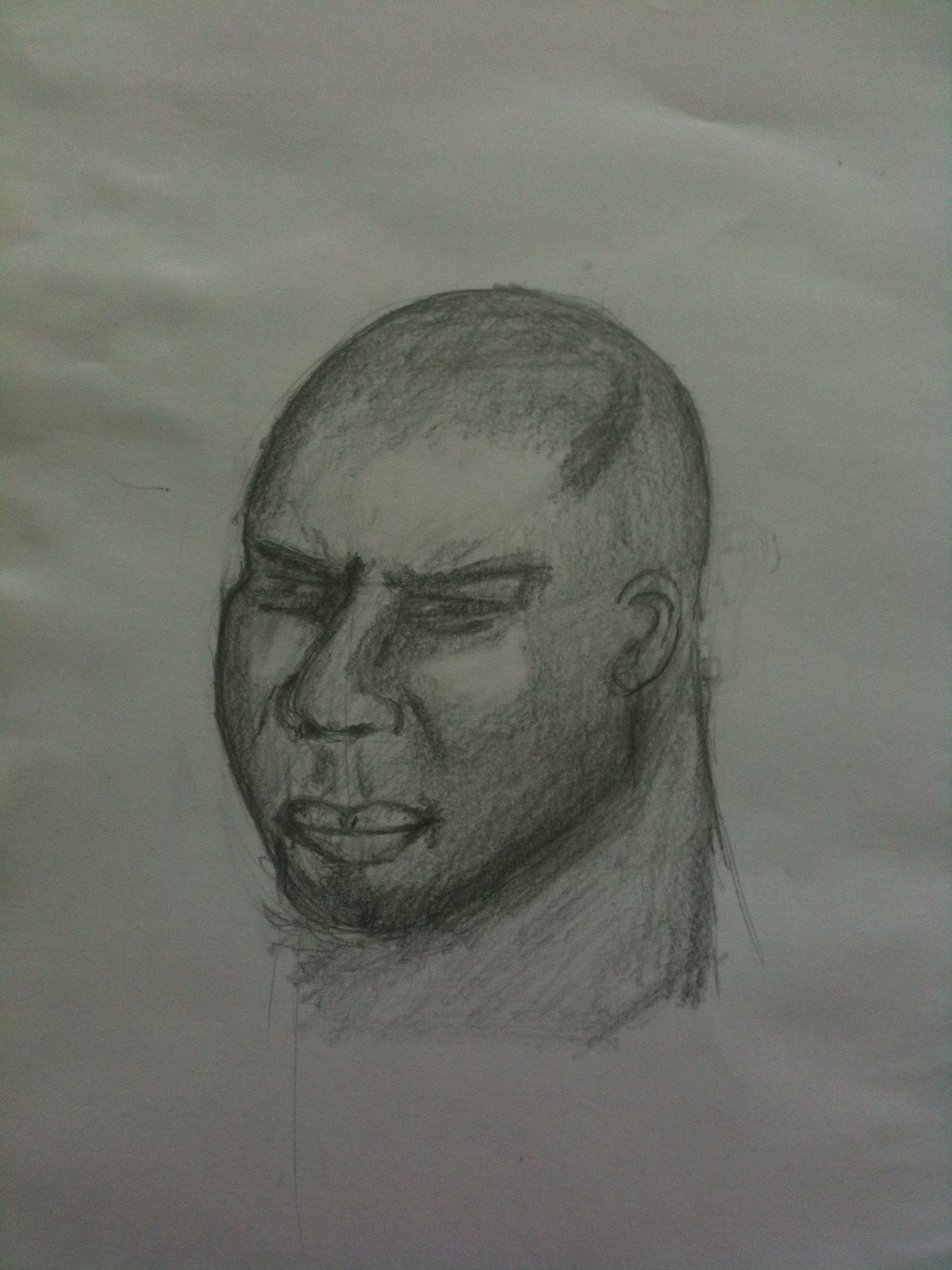This detailed black-and-white pencil sketch depicts the head of a man with predominantly bald features. The artist has skillfully used shading to represent light reflection or possible stubble on the scalp. A striking detail is a singular tuft of hair, carefully drawn, that loops forward toward the forehead. The man's face is marked by squinted eyes with dark pupils, a prominent nose meticulously rendered at the tip, and a large mouth that emphasizes a pronounced jawline. His expression conveys a sense of anger or seriousness. The sketch extends down to include some shading on the neck. The drawing is on a slightly crumpled piece of white or off-white paper, which gives the surface a wavy texture. The background behind the paper is not visible.